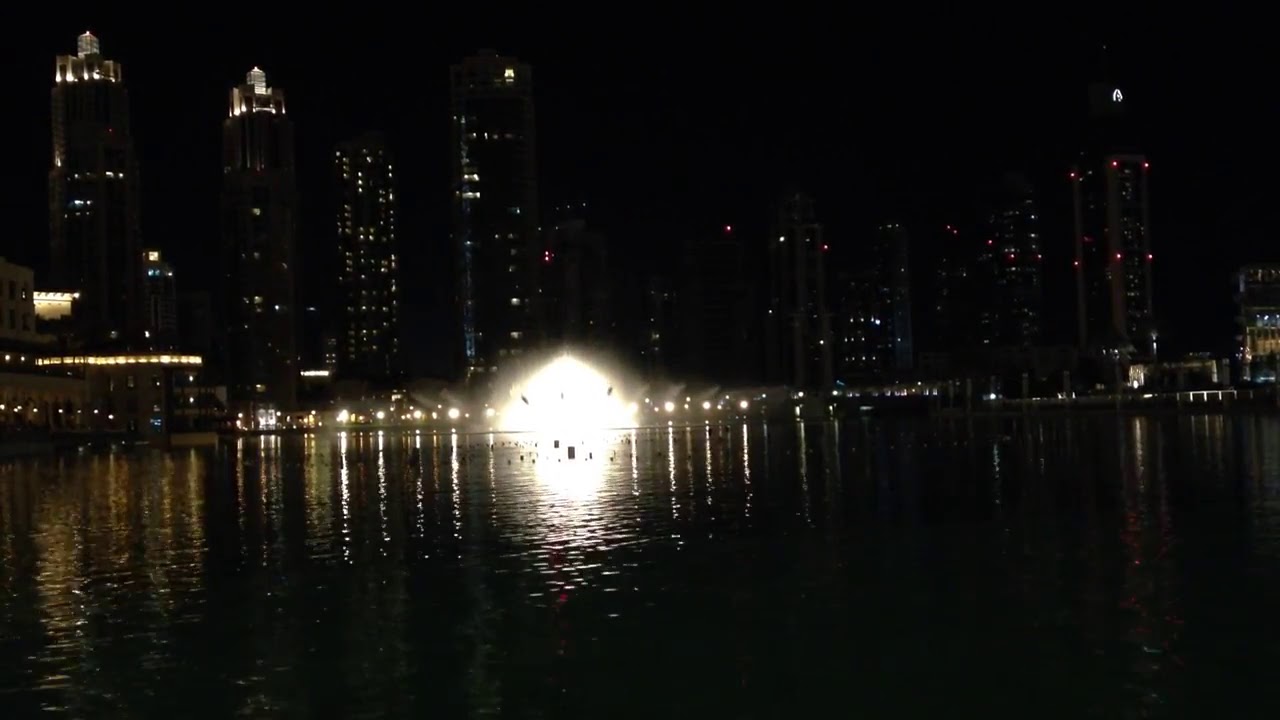A nighttime scene showcasing a large metropolis with a dark sky overhead and a city skyline composed of tall, illuminated skyscrapers. The buildings feature a mix of white, bluish, pink, and yellow lights shimmering from top to bottom. In the foreground, there is a vast body of water with a mixture of dark black and steel gray hues, mirroring the vivid lights of the city. Right at the center of the image, a bright, dome-shaped flash of light, resembling a small explosion, illuminates the water, casting orange and yellow reflections and creating a notable spectacle. Along the water's shore, additional lights line up to the left and right of the central flare, while some smaller buildings, only a few stories high, are visible to the left side of the scene. Also observed in the water are ripples and scattered black specks, adding depth and texture to the reflective surface. In the tranquil river, there are small boats docked, enhancing the serene yet vivid ambiance of the cityscape.